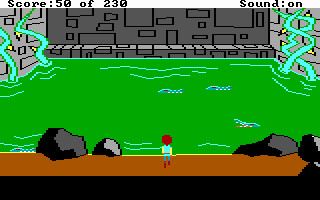Screenshot from an old video game, likely from the late 1970s or early 1980s. In the image, a boy or young man, with reddish-brown hair, stands on a patch of dirt. He is wearing an aqua blue vest and has yellow sleeves. In front of him is a green pool of acid with several tentacles protruding from it. A rocky path is visible nearby, and beyond the acid pool stands a castle wall. The scene implies that the character is attempting to reach the castle wall but is obstructed by the hazardous acid pool. In the top left corner of the screen, the score is displayed as "50 of 230".